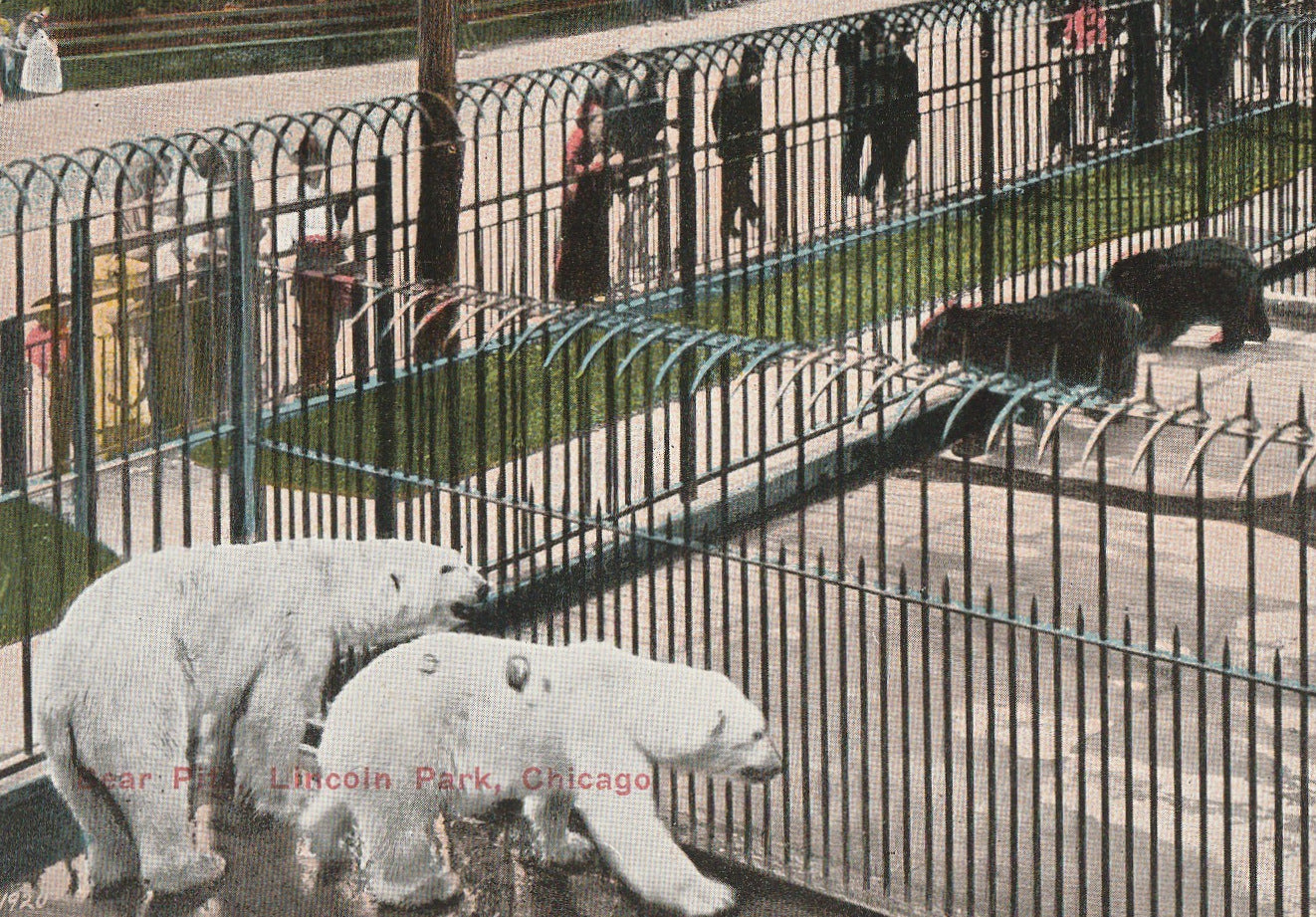This horizontal rectangular photograph, seemingly from the early 1900s, appears to have been colorized digitally, retaining some misaligned hues and a grainy quality characteristic of older images. It captures a zoo enclosure at Lincoln Park Zoo in Chicago. In the foreground on the left, two large polar bears occupy a caged setting. There are visible spikes on the fencing between enclosures. To the right, in a separate enclosure, two brown bears are present. The lower-left corner above the polar bears features light pink text that reads "Bear Pit, Lincoln Park, Chicago." A grassy area and a sidewalk span the space in front of the bear enclosures, leading up to a taller metal fence beside which numerous zoo patrons, men and women, are seen observing the bears. Behind them stretches a wide walkway, flanked by more grass and a potential sitting bench.